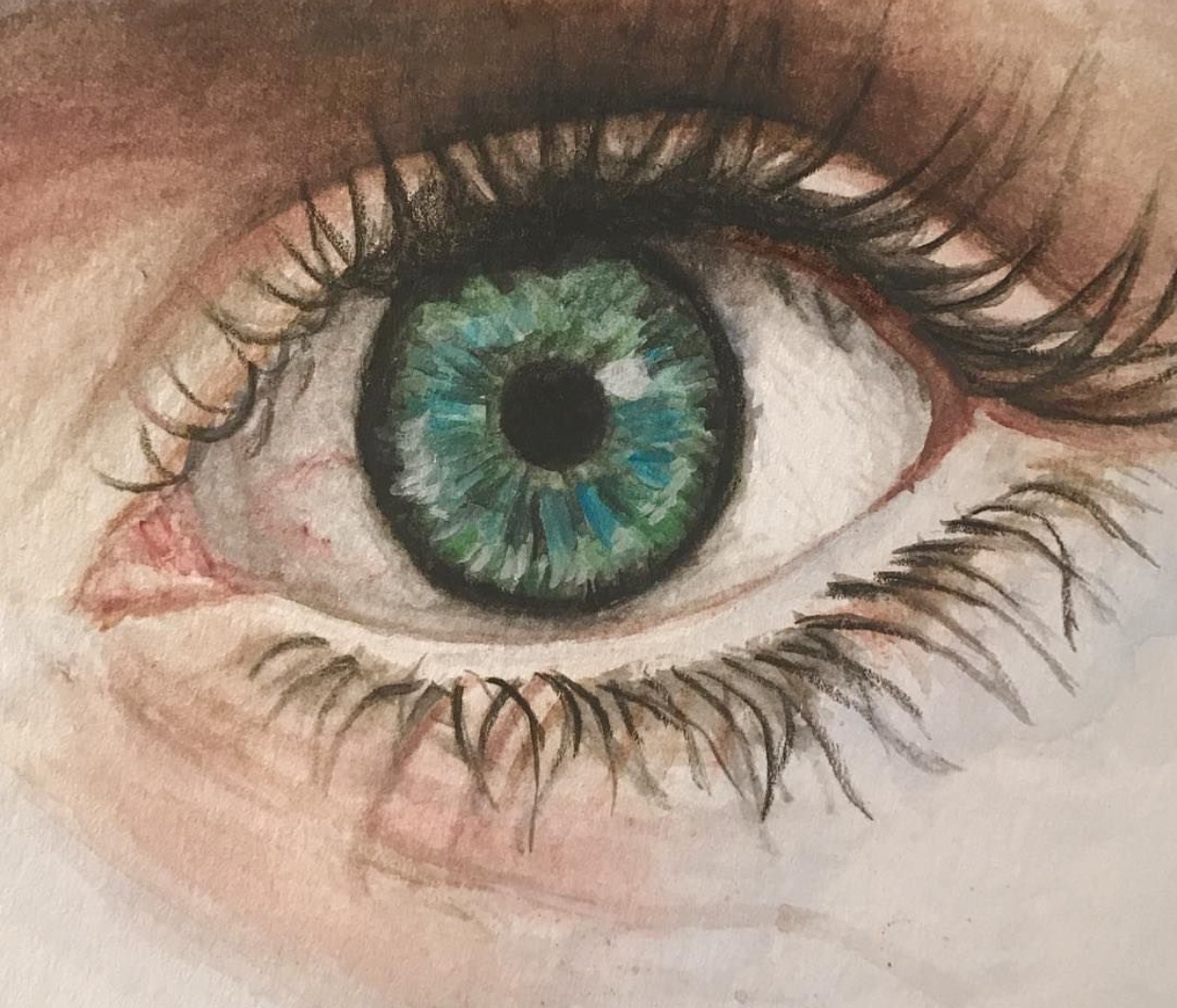A detailed and artistic sketch captures the close-up of a feminine eye belonging to a fair-skinned person. The eye features a mesmerizing blue-green iris, sharply contrasting with the dark black pupil and the white sclera. Long, dark lashes—accented with mascara—frame the eye, with the upper lashes appearing especially prominent. The lower lashes are distinctly black, adding to the eye's expressive look. Dark eye shadow, or perhaps a shadow effect from the sketch, accentuates the area above the eye. Fine lines under the eyelid suggest a hint of age or emotion, adding depth to the composition. The overall effect is both striking and evocative, emphasizing the intricate details that make the eye a focal point of human expression.